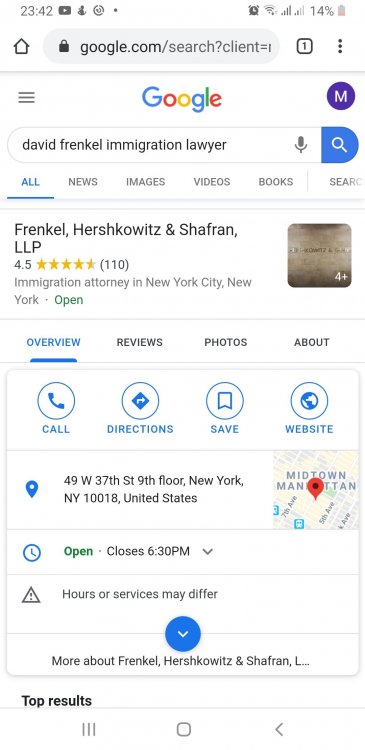The screenshot captures the display of a phone at 23:42 with 14% battery remaining. The web address in the address bar reads "google.com/search?client=" and beneath it lies a search box with the query "David Frenkel immigration lawyer." Adjacent to the search box are a microphone icon and a magnifying glass icon. Below the search results, the first entry highlights "Frenkel, Hershkowitz, and Schifron, LLP," rated 4.5 stars based on 110 reviews. It's identified as an immigration attorney firm located in New York City, New York. The listing indicates the firm’s available status with options for users to view "Overview," "Reviews," "Photos," and "About."

Additional action buttons for "Call," "Directions," "Save," and "Website" are presented. A blue location pin followed by the address "49 West 37th Street, 9th Floor, New York, New York, 10018, United States" is shown. The firm is marked "Open," with closing time at 6:30 PM. A disclaimer follows, noting that "Hours of service may differ."